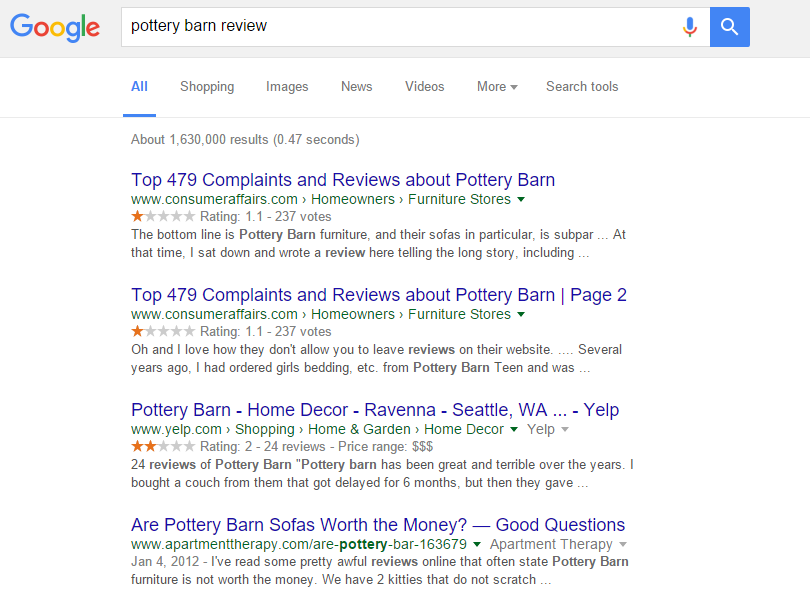This is a detailed screenshot of a Google search results page. At the top, the iconic Google logo is prominently displayed next to the search bar where the query "Pottery Barn Review" has been entered. The search yielded approximately 1,630,000 results. The top four search results are shown prominently below the search bar. The first two results are from ConsumerAffairs.com, the third result is from Yelp.com, and the fourth is from ConsumerAssuranceTherapy.com. Above these results, there are several filtering options including "All," "Shopping," "Images," "News," and "Videos," with an additional "More" dropdown menu for further filtering options.